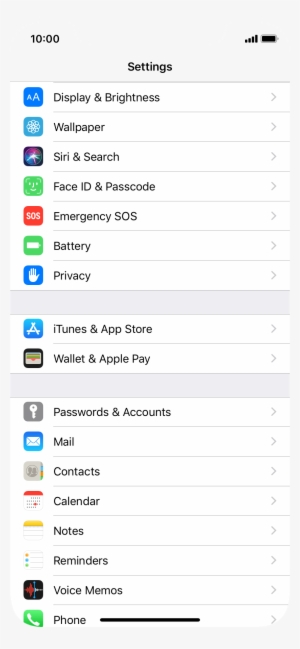The image showcases a cell phone screen displaying the settings page. Positioned at the top left corner, the time reads 10:00, while the top right corner features a wireless icon and a nearly full battery icon. The page title "Settings" is displayed prominently at the top. A vertical column of icons, each representing different settings options, is arranged on the left side.

The first icon, a blue square containing two white "A" letters, is labeled "Display & Brightness." Below it is another blue icon with a unique design, labeled "Wallpaper." Next, there's a black square with "Siri & Search" written beside it. Following that is a green icon with a smiley face labeled "Face ID & Passcode." The subsequent icon is red, labeled "Emergency SOS."

A green icon with a white battery symbol is labeled "Battery." Further down, a blue square with a hand icon is labeled "Privacy." Below this, another blue square with the letter "A" represents "iTunes & App Store." Next is a black square with an image resembling a payment card, labeled "Wallet & Apple Pay." Continuing down, a gray square with a key icon represents "Passwords & Accounts." A blue square with an envelope icon is labeled "Mail." 

Moving further, a gray square with two people icon is labeled "Contacts," followed by an icon of a calendar labeled "Calendar." An icon resembling a notepad labeled "Notes" comes next, followed by an icon of a sheet of paper with lines labeled "Reminders." A black icon labeled "Voice Memos" is next in line, and the final icon in this column is green with a white phone symbol, labeled "Phone."

The visually organized layout and distinct iconography make it easy for users to navigate the settings on this device.